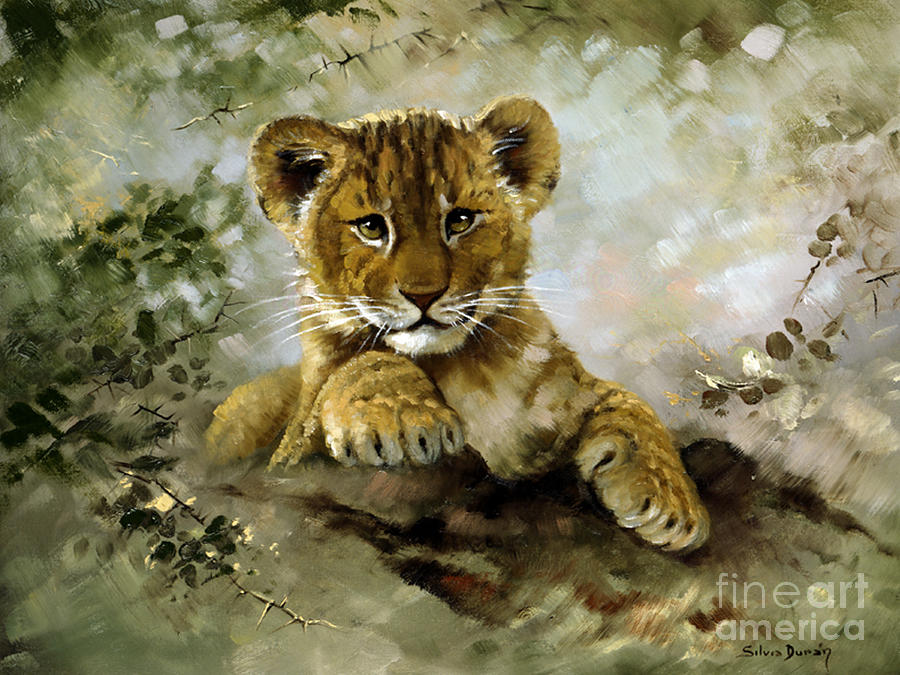This image showcases a charming piece of art, prominently featuring a small lion or tiger cub, rendered with what appears to be crayon. The cub, depicted in warm shades of orange and orangey-brown, sits facing the viewer, exuding an endearing innocence. Its circular, fluffy ears perch atop its head, contributing to its playful appearance. Bright white whiskers adorn its face, complementing a black, cheerful smile that contrasts with the white rims encircling its vibrant green eyes. The cub's front paws, detailed with black nails, are clearly visible, while its back and hind feet are subtly obscured behind its head, chest, and front paws. Adding to the natural ambiance, lush green bushes surround the cub, enhancing the overall composition. In the bottom right corner of the artwork, the words "Fine Art America" are inscribed in white letters.